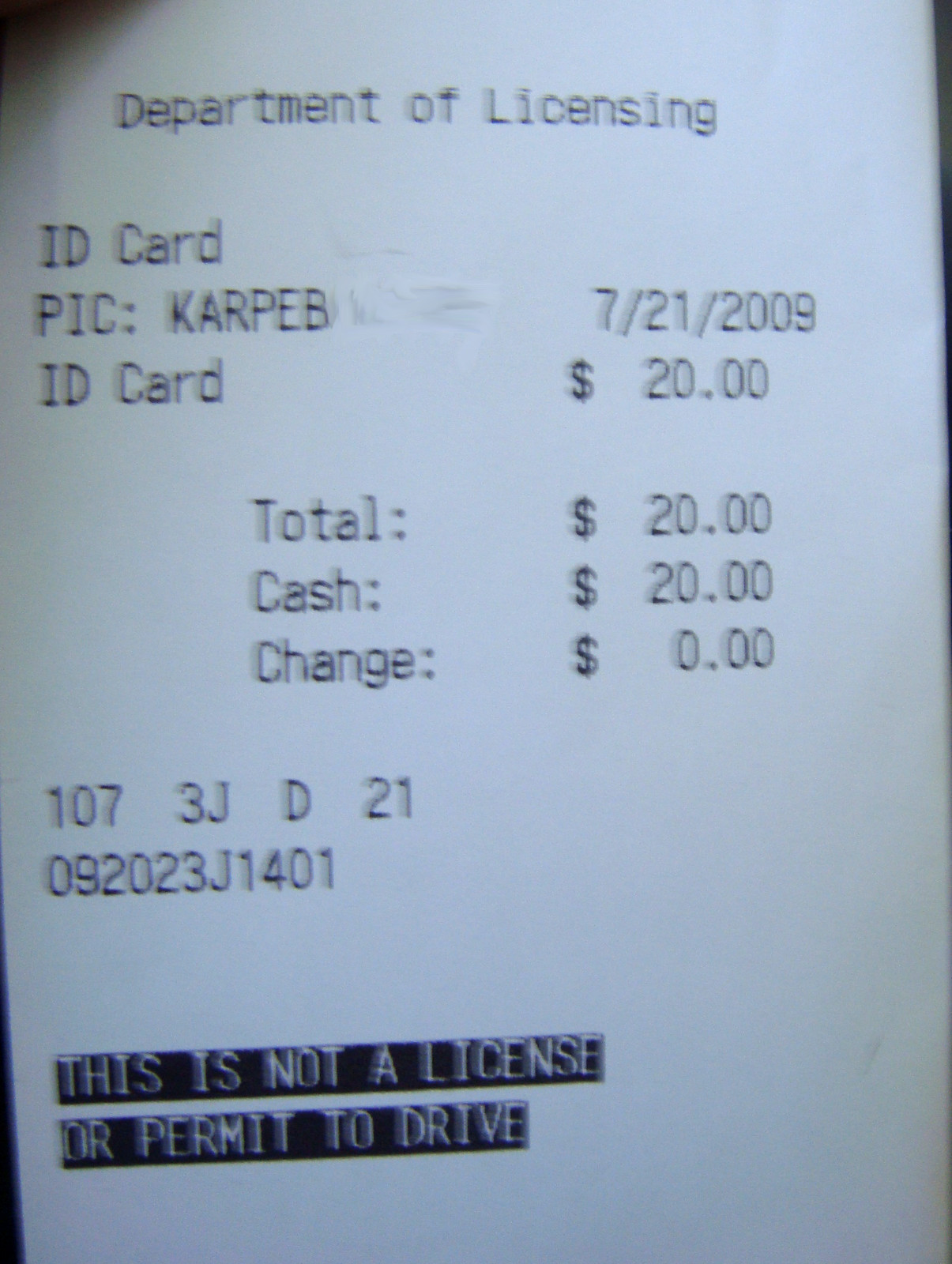The image displays a detailed paper receipt from the Department of Licensing. At the top of the white receipt, printed in black font, is the heading "Department of Licensing." Directly below, it indicates "ID Card" followed by "PIC: K-A-R-P-E-B." The date "7-21-2009" is shown next to it. On the left, beneath the PIC label, it states "ID Card," with "$20.00" detailed to the right, marking the charge for the ID card. Below this, the receipt lists "TOTAL: $20.00," "CASH: $20.00," and "CHANGE: $0.00" in a similar layout, with the amounts aligned to the right. Alongside other details, such as the numbers "107 3J D 21" and "092023J1401" near the bottom left, the most striking feature lies at the bottom of the receipt. It has a black highlighted background with white text declaring, "this is not a license or permit to drive." The repetitive confirmation of the cash payment amount and zero change emphasizes the transaction's completion.